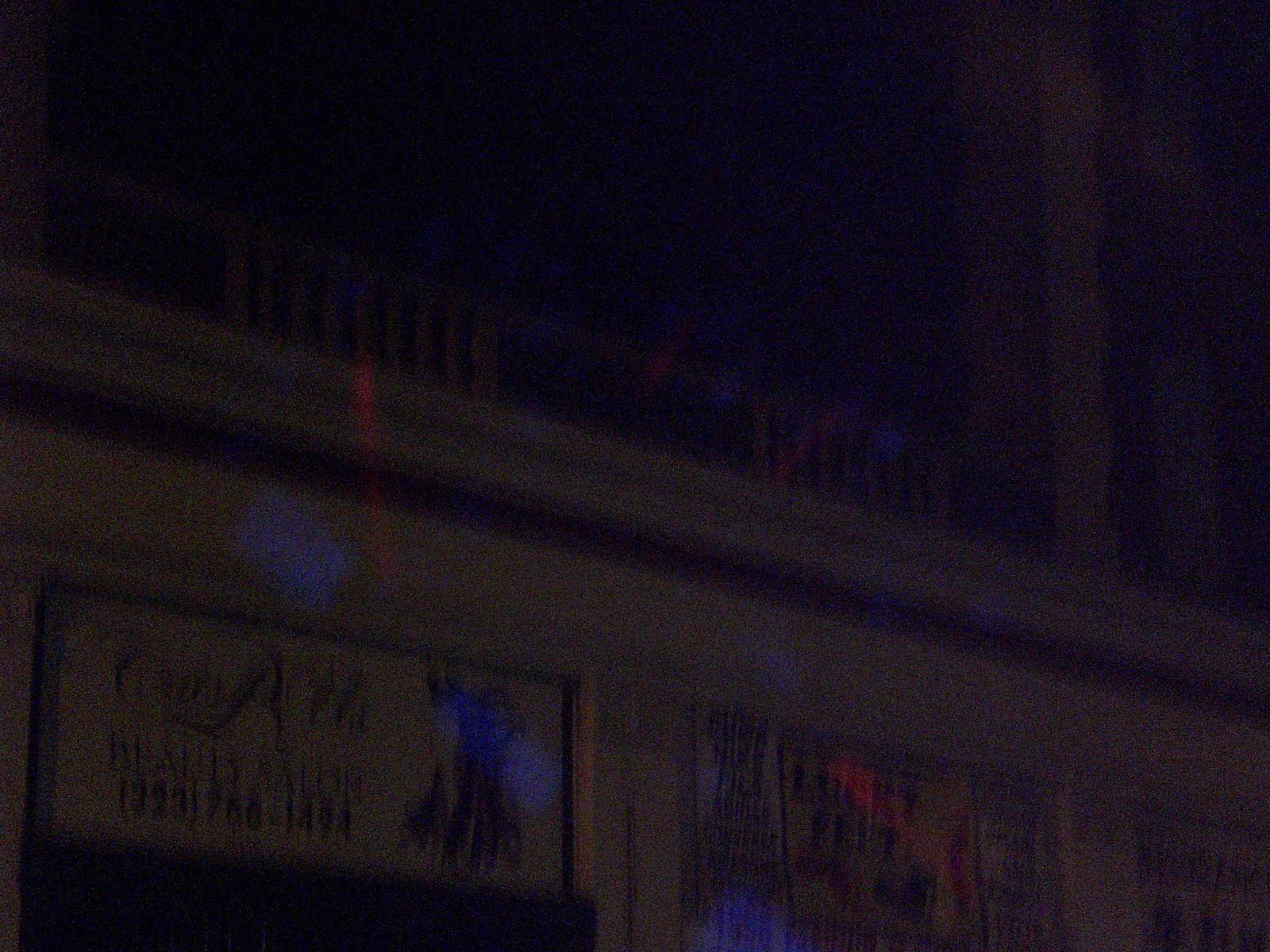In this image, a blurry and dark photograph captures the front facade of a building at night. Blurry and haloed lights, emitting bluish and reddish hues, obscure the visibility of the signage. At the center, one of the signs barely legibly reads "Beauty Salon," followed by a phone number that appears to be 323-256-1491 or 323-266-1494. Adjacent to it, another sign seemingly advertises "Lucky Fruit," although the full details are obscured by the poor image quality. Above the signage, a structure resembling a grate or railing—similar to a heating duct register—adds to the indistinctness of the scene. The overall dimness and blur make further identification challenging.